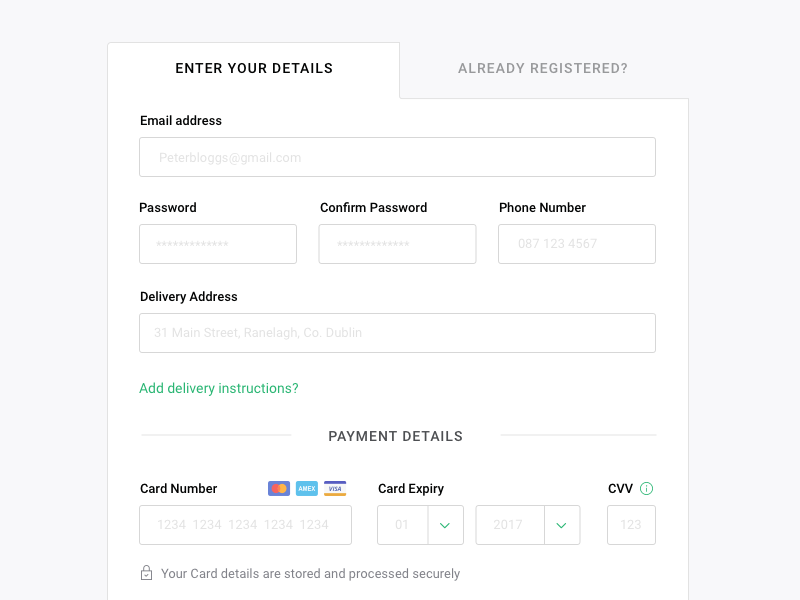The image depicts a detailed registration and payment form with the following sections and placeholders:

1. **User Registration Details**:
   - **Email Address**: Input field with the placeholder text "peterblogs.gmail.com".
   - **Password**: Input field with masked characters displayed as asterisks.
   - **Confirm Password**: Input field with placeholder text displaying more asterisks.

2. **Contact Information**:
   - **Phone Number**: Input field with placeholder "087-123-4567".
   - **Delivery Address**: Input field filled with "31 Main Street, Ranoco, Dublin".
   - **Delivery Instructions**: An input section with a question mark prompting for additional instructions.

3. **Image Upload Section**: An area where users can upload images related to their registration.

4. **Payment Details**:
   - The form is divided into left and right sections, with specific details required for card payment.
   - On the very bottom left:
     - **Card Number**: Placeholder text "1234 1234 1234 1234".
     - **Accepted Cards**: Discovery, Visa, and American Express logos indicated.
     - **Expiration Date**:
       - Drop-down menus for the month (placeholder "01") and year (placeholder "2017").
     - **CVV**: Input field with placeholder "123".

5. **Background**: The background is predominantly white, highlighting the different sections and input fields.

6. **Security Message**: A note at the bottom assures that "Your card details are stored and processed securely."

The form is meticulously designed, providing clear placeholders and secure input fields for user convenience and protection.